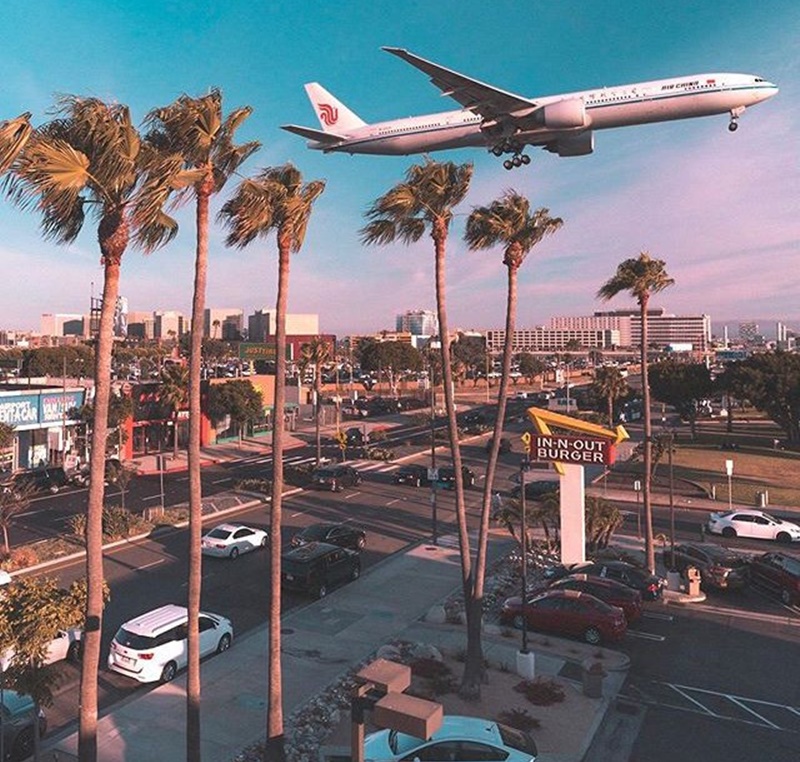The photograph captures an urban scene taken from a slight elevation, likely a few stories up, overlooking a bustling city that could be Los Angeles or Phoenix. In the bottom right corner, there's a parking lot filled with numerous cars, adjacent to a prominent In-N-Out Burger sign with a yellow arrow pointing to the right. To the left of the parking lot, a main road is busy with traffic moving in both directions, with a particularly noticeable white van on the bottom left. Alongside the road and in front of the parking lot stand tall palm trees, adding a touch of greenery to the cityscape.

Across the street from the parking lot, additional lanes of traffic flow parallel to more distant buildings and structures. The skyline is dotted with taller buildings, suggesting a well-developed urban area, and further punctuated by more sporadic trees. A striking feature of the image is a large passenger jet flying low overhead, with its landing gear deployed, indicating it's either approaching for a landing or just taken off. The jet is predominantly white, adorned with a blue stripe running its length and a red logo on the tail fin. The sky is a vibrant blue with a few clouds, tinged pink, hinting at either sunrise or sunset, creating a picturesque backdrop for the scene.